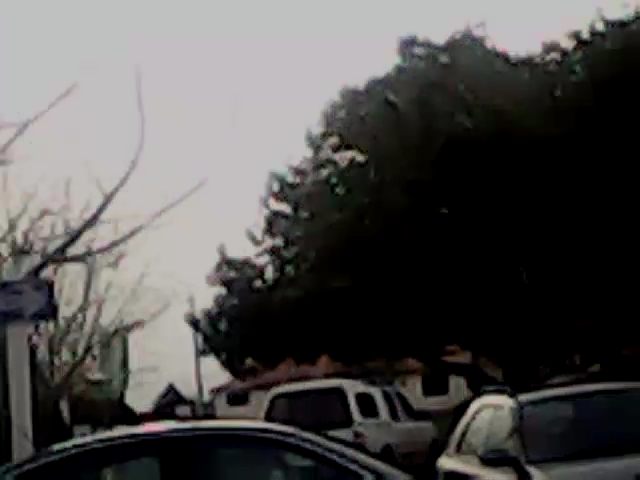This daytime photograph, slightly blurry and tilted to the left, presents a landscape orientation. In the foreground, the tops of two vehicles are visible. The vehicle on the left shows part of its left side, displaying only the upper portions of its windows and roof, while the one on the right reveals more details including the hood, windshield, right-side rearview mirror, and double windows. Situated behind these two vehicles sits a white pickup truck with a camper shell on its bed, resting under the shade of a sprawling tree. Further into the background, a building is present, partially obscured by the large tree in front of it. On the left side of the image, an edge of a street sign pointing to the right is visible. The scene is complemented by several scrub-type trees and an overcast sky looming in the background.